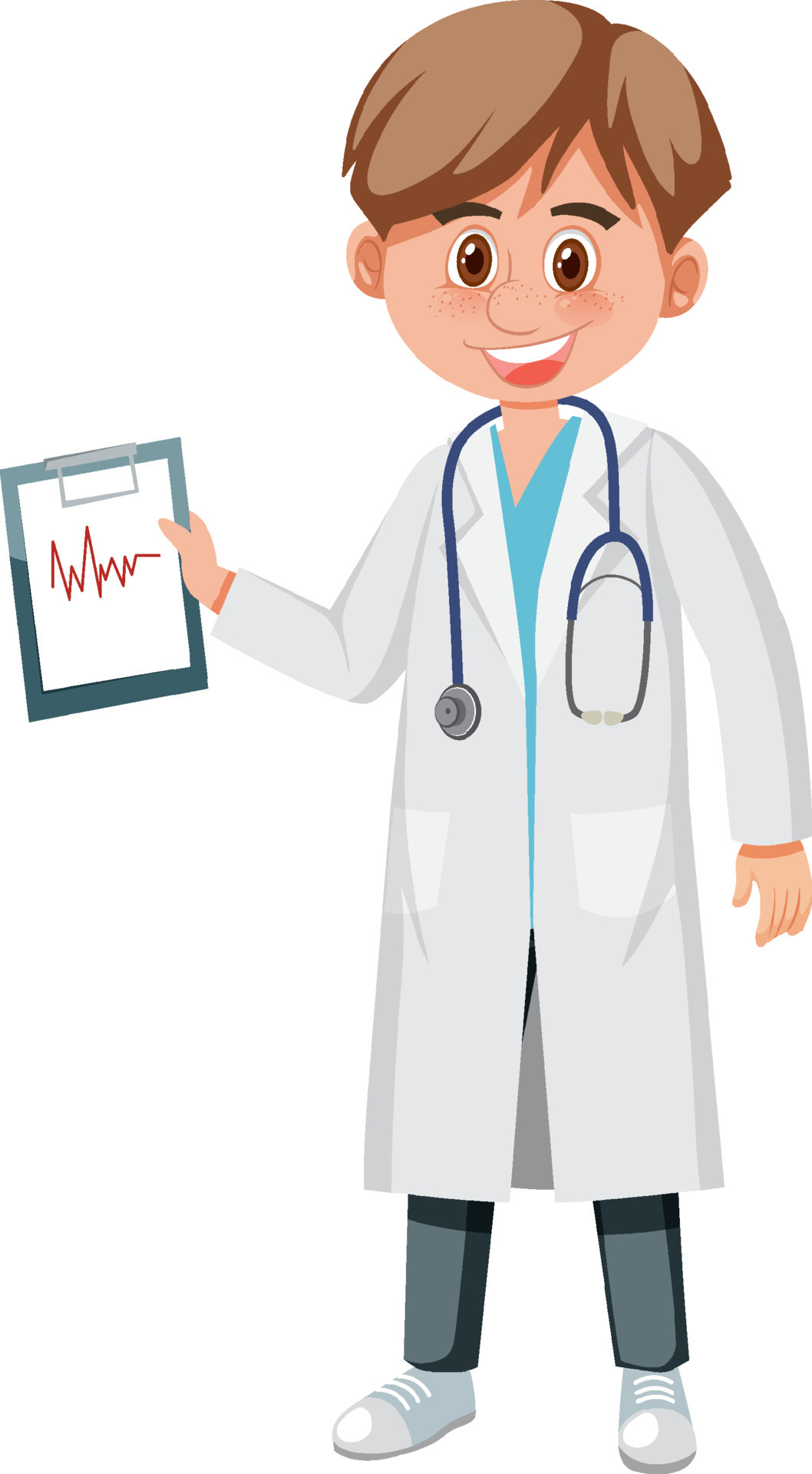This image depicts a young, cartoon-style male doctor standing against a white background. He has short brown hair, brown eyes with black eyebrows, and freckles on his cheeks, giving him a youthful, cheerful appearance emphasized by his large smile. He is dressed in a professional medical outfit consisting of a long white lab coat over light blue scrubs, visible through the V-shaped neckline of the coat, and dark gray pants. On his feet, he wears white sneakers. Around his neck is a dark blue stethoscope with silver accents. In his right hand, he holds a clipboard featuring a white sheet with a noticeable red jagged line, reminiscent of seismographic or heart rate monitor readings. The drawing employs a simplistic, minimalist art style without any outlines, enhancing the cutesy charm of the character.